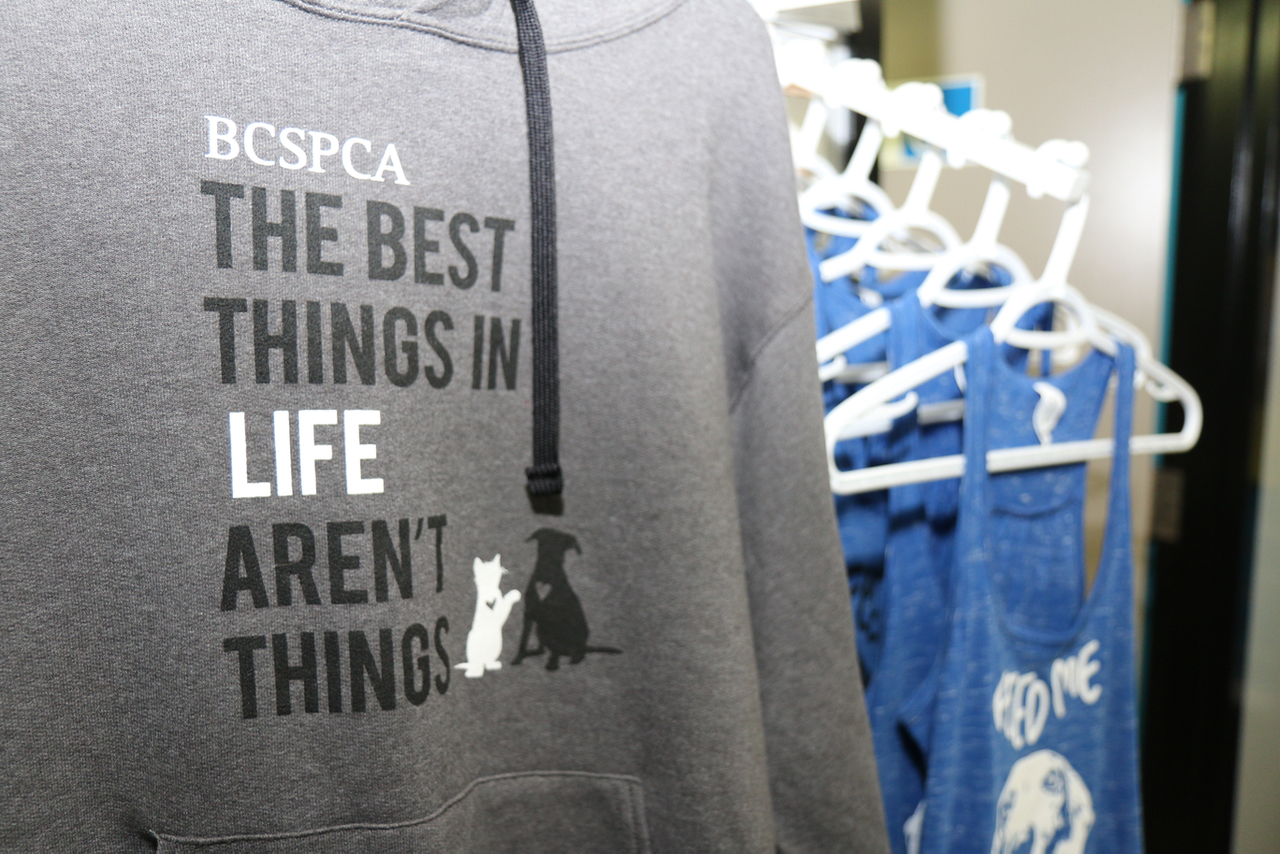The image shows a close-up of a gray hoodie or sweatshirt dominating the left side, taking up more than two-thirds of the frame. This hoodie features a black drawstring and a print of a white cat and a black dog with heart-shaped cutouts around their necks. Above the image of the animals, in white text, it says "BCSPCA." Following below, the text reads in alternating black and white fonts: "The Best Things in Life Aren't Things." Behind the hoodie, hanging diagonally on a white rod, are several blue sleeveless shirts on white hangers. The front shirt displays a white graphic with the words "Feed Me" above a depiction of what appears to be an animal's face. The background is minimal and the emphasis is on the clothing items.